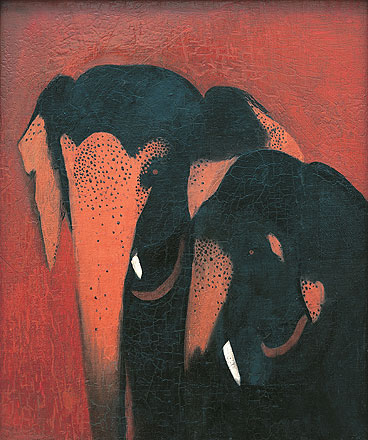This is a semi-realistic oil on canvas painting featuring two elephants side-by-side. The elephants exhibit a unique color palette with orange ears, trunks, and eyes, contrasted against their black heads and bodies. Each elephant has a visible white tusk, and they appear to be touching, with one's left ear touching the other's right ear. The surface of the painting shows cracks, contributing to an aged, textured appearance. In the background, a mix of deep, muted burgundy, burnt brownish-red, and hints of gray provides a dynamic, almost volcanic texture. The crimson hues are particularly intense toward the top, resembling a lava-like texture, and lower-left sections show signs of dripping or scraping, likely applied with a palette knife. The elephants' small, visible eyes and distinct, tusked faces stand out against the richly colored background, giving the artwork an old world yet evocative style.